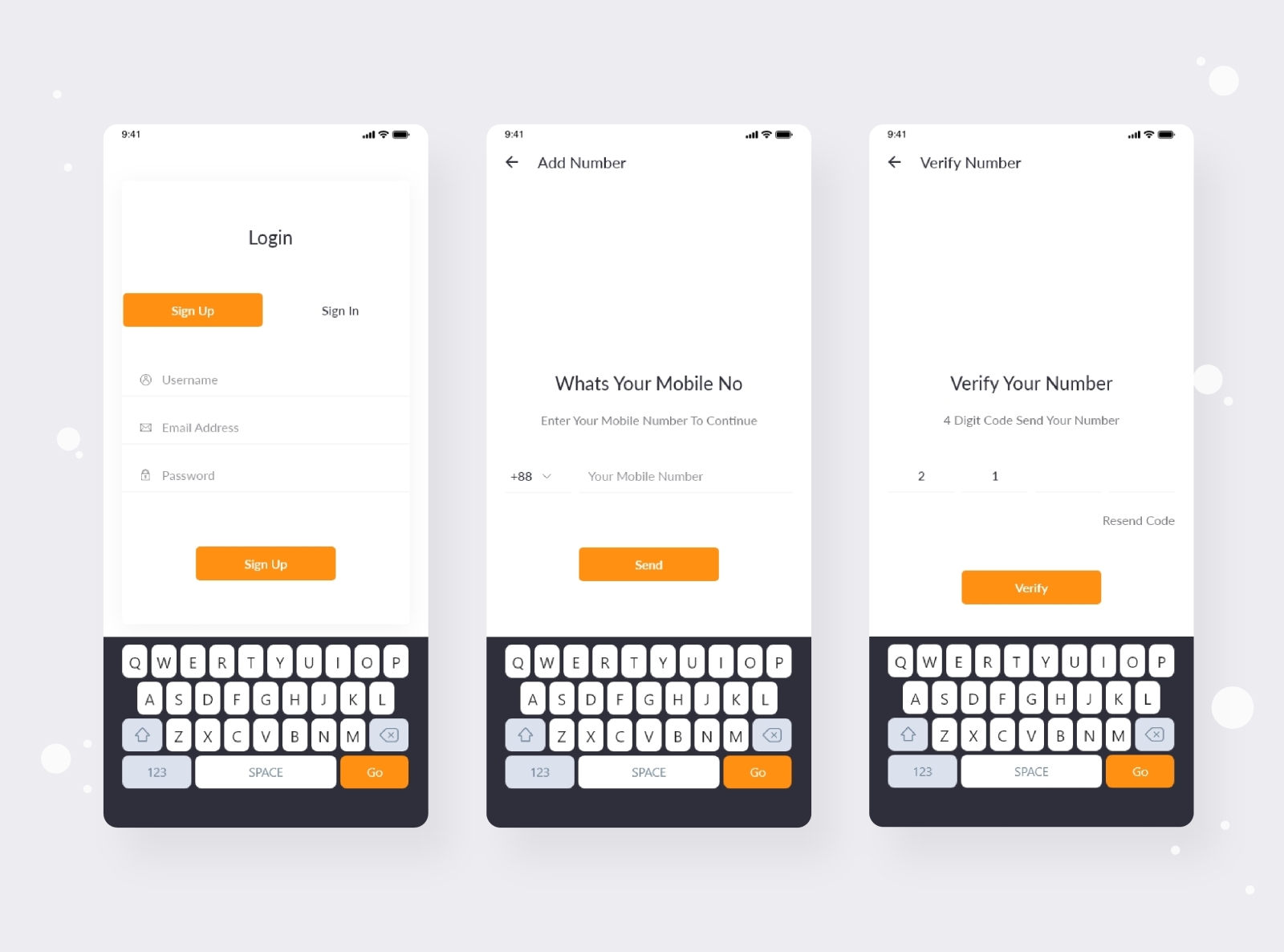This image displays three sequential mobile screenshots from the same app, showcasing the user flow from login to number verification. 

- **First Screenshot (Left):** This is the **Login Page.** It features two distinct buttons: a prominent sign-up button in **orange** and a sign-in button in **white with black text.** The page contains three input fields, each accompanied by an icon, for **Username, Email Address,** and **Password.** Additionally, there is an **orange sign-up button** with white text situated at the bottom center of the page. Below this, an on-screen **QWERTY keyboard** with a black background and white keys is displayed, featuring an **orange 'Go' button** in the bottom right corner.

- **Second Screenshot (Middle):** This page follows the same design format as the first but introduces an additional section. The headline reads, **"What's your mobile number?"** Users are prompted to enter their mobile number in a designated input box. The virtual keyboard remains visible at the bottom, consistent with the first screenshot.

- **Third Screenshot (Right):** This page is for **Number Verification.** It instructs the user to **"Verify your number"** by entering a four-digit code sent to their mobile number. An **orange 'Verify' button** is prominently placed above the virtual keyboard, which remains consistent with the previous screenshots.

These screenshots collectively guide the user through the initial steps of account creation and verification in a streamlined and visually cohesive manner.